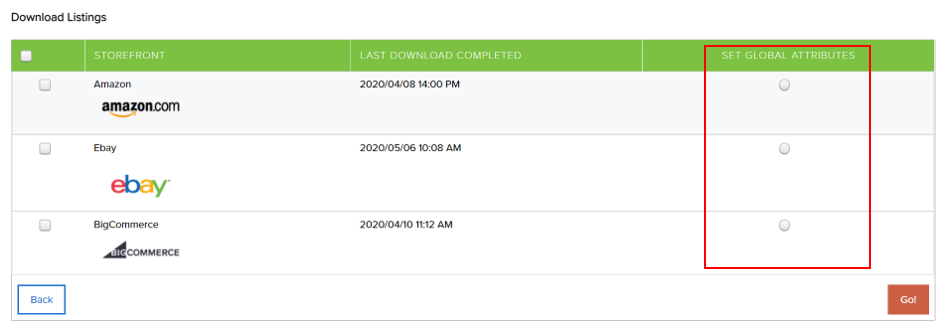This image is a screenshot of a download management interface, likely from a software application used to track downloads from various online storefronts. The image is in a landscape orientation without any defined outside borders, approximately two to three times longer than it is tall.

At the top, there is a prominent black box or text that reads "Download Listings." Beneath this, a gray header spans horizontally across the screen, divided into different categories by thin white lines. The categories listed are, from left to right: an empty gray checkbox, "Storefront" written in white font, "Last Download Completed" also in white font, and finally "Set Global Attributes."

Directly below this header, three long horizontal boxes are displayed, separated by thin gray lines. Each box pertains to a different online storefront, containing the following information:

1. **Amazon**: The first box has an empty checkbox on the left, followed by the text "Amazon" and the Amazon logo. The "Last Download Completed" date is listed as "4-8-2020 at 14:00," and the "Set Global Attributes" option is unchecked.

2. **eBay**: The second box follows a similar format with an empty checkbox, the text "eBay," and its logo. The "Last Download Completed" date is "5-6-2020 at 10:08," with the "Set Global Attributes" option also unchecked.

3. **BigCommerce**: The final box contains an empty checkbox, the text "BigCommerce," and its logo. The "Last Download Completed" date is incorrectly formatted as "4-10-2020 at 11:12-2020," possibly indicating a typo. The "Set Global Attributes" option remains unchecked across all entries.

A vertical red box encompasses all the entries, drawing additional attention to this section of the interface.

This detailed interface ensures users can monitor and manage their download activities across multiple online storefronts efficiently.